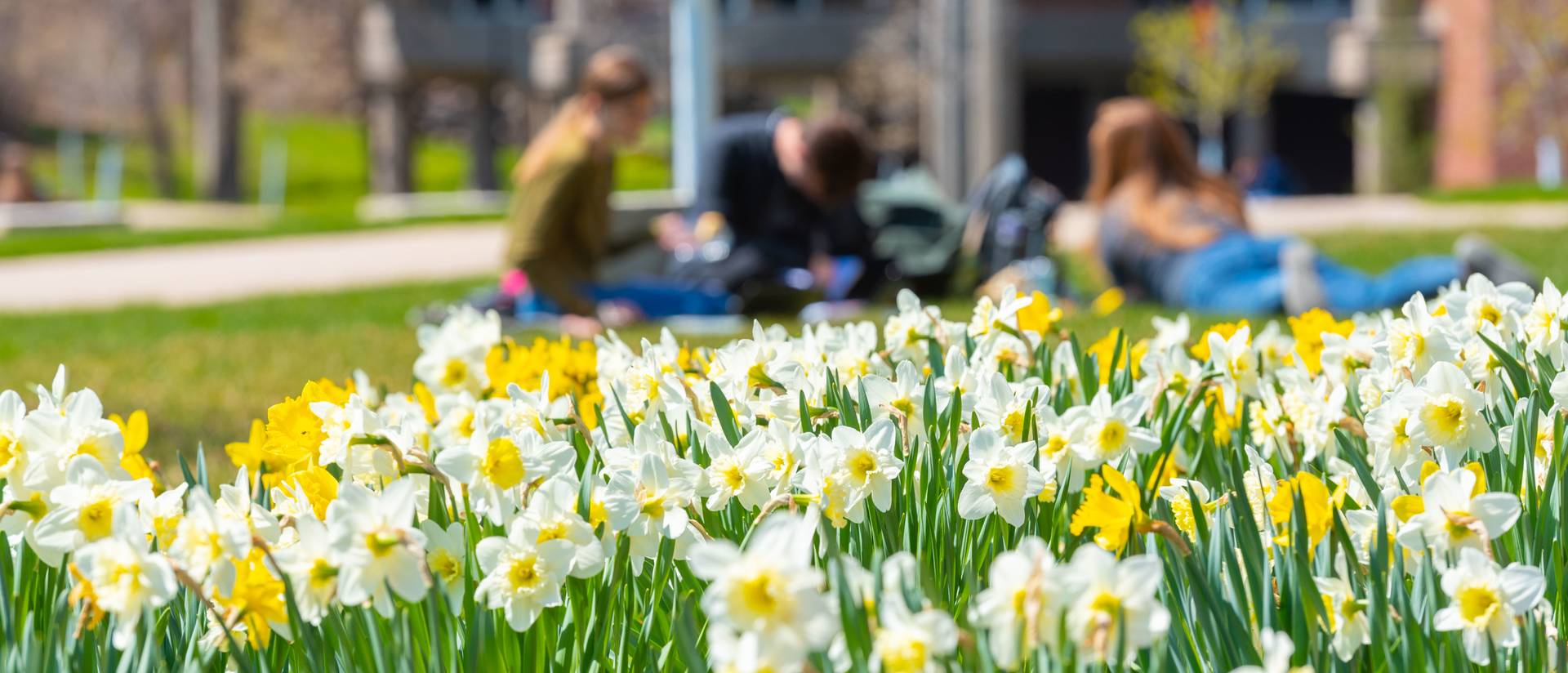The image captures a vibrant, sunlit scene on what appears to be a college campus. The foreground is dominated by a large patch of blooming lilies, which are either entirely yellow or white with yellow centers. These flowers stretch across the width of the image, their green stalks and leaves standing vividly against the ground. Just beyond the flowers, three students are sprawled out on a lush green lawn, slightly out of focus, suggesting a casual, relaxed atmosphere.

The group consists of one girl and two boys, hinting at a break between classes. They all have backpacks nearby, reinforcing the student theme. The girl, positioned on the right, is wearing blue jeans and a gray shirt. The boy next to her, in the center, is dressed in a black top and darker jeans. The boy on the left wears blue jeans and a gold-colored top. From this low-angle perspective, you can see a sidewalk running laterally behind them, and several indistinct campus buildings form the background.

The scene is bathed in daylight, with the sun high in the sky, suggesting it’s either late morning or early afternoon. Overall, the image evokes a serene moment of reprieve for the students amidst their academic day.